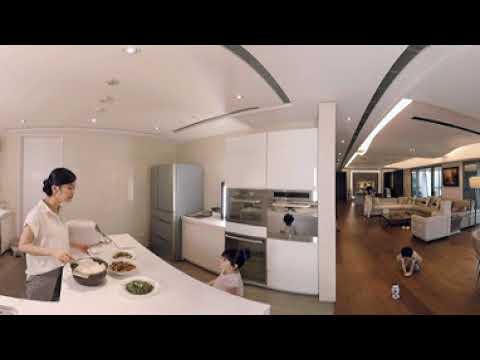In this image, taken through a fisheye lens that distorts the scenery, a woman is seen standing in a white kitchen on the far left side. She appears to be of Asian descent, with black hair tied back in a bun. She is wearing a white shirt that reaches just below her elbows and gray pants. The woman's hands rest on the counter in front of her, where she is preparing food. There are four bowls placed on the counter: a gray bowl containing white food directly in front of her, which she appears to be using utensils with, and three other bowls—one white, one with green food, and one with brown food.

Opposite the woman, a child stands on their side of the counter, wearing a pink shirt with black hair that reaches nearly to the counter's top. Behind the child, the kitchen features a silver refrigerator, a silver oven, a microwave, and white cabinets. The back wall of the kitchen is white, with a white door visible on the back left side behind the woman. The ceiling has round lights and gray stripes. The floor in the kitchen area is gray, while transitioning to wooden in the adjoining living room space.

In this living room area to the right, a young child with black hair is kneeling on the wooden floor, attentively playing with a small white animal. The living room is furnished with a gray couch, and a window at the back allows some green and white light to filter through, adding to the room’s ambiance. The fisheye lens creates a slight separation between the kitchen and the living room, making the layout appear somewhat surreal, almost like a cinematic set.